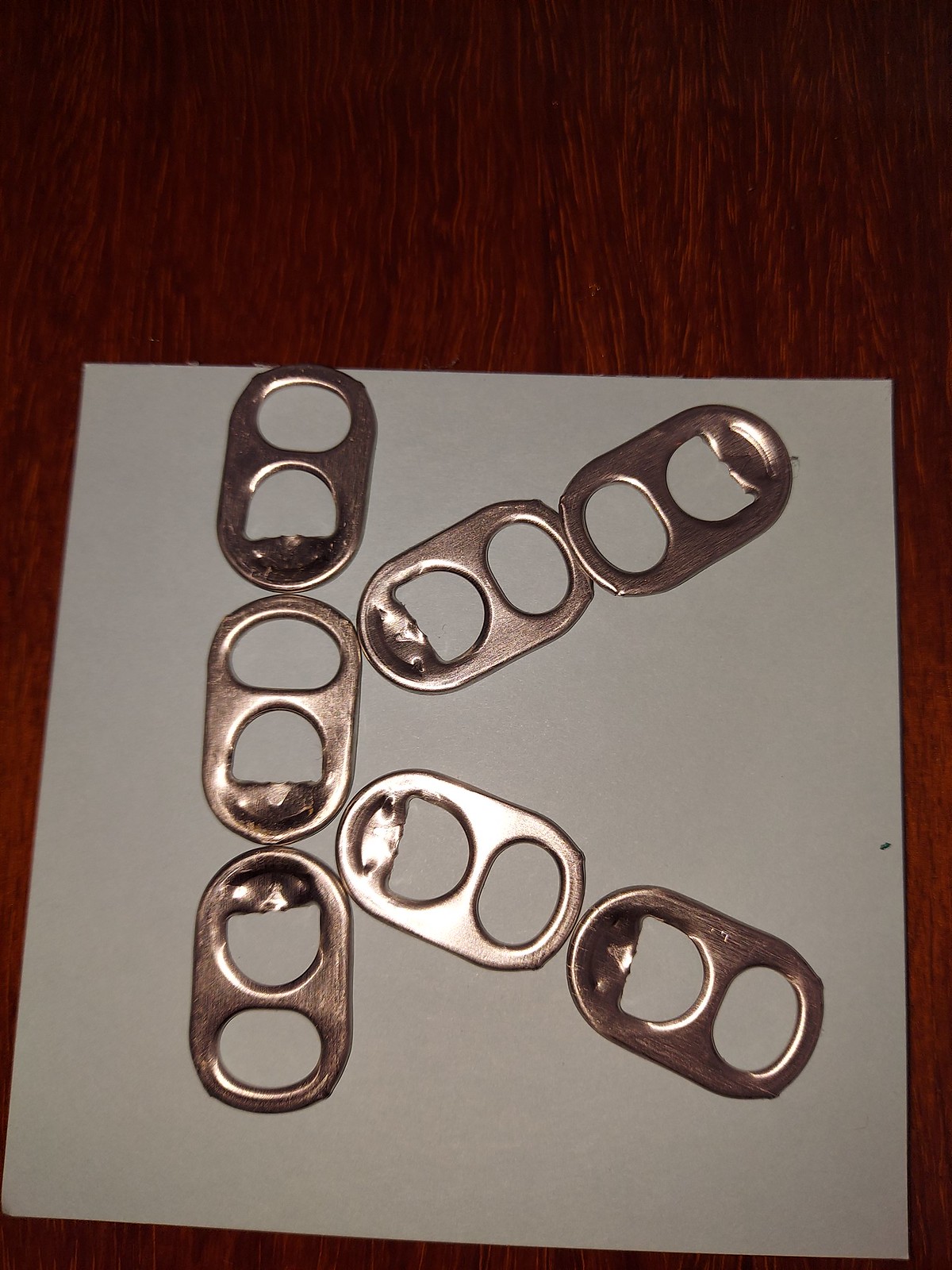The image depicts a dark red-brown, textured wooden table with a small, square piece of light-colored paper placed on it. On the paper, seven shiny silver can pull tabs are meticulously arranged to form the letter "K". Three of these tabs are aligned vertically to create the backbone of the letter, while the remaining four tabs are positioned at angles to complete the "K" shape—two tabs angled up to the left and two angled down to the right. A tiny black speck is noticeable on the far right-hand side of the paper, adding a minor detail to the composition. The lighting in the image is somewhat dim, with a subtle reflection of light off one of the shiny pull tabs.